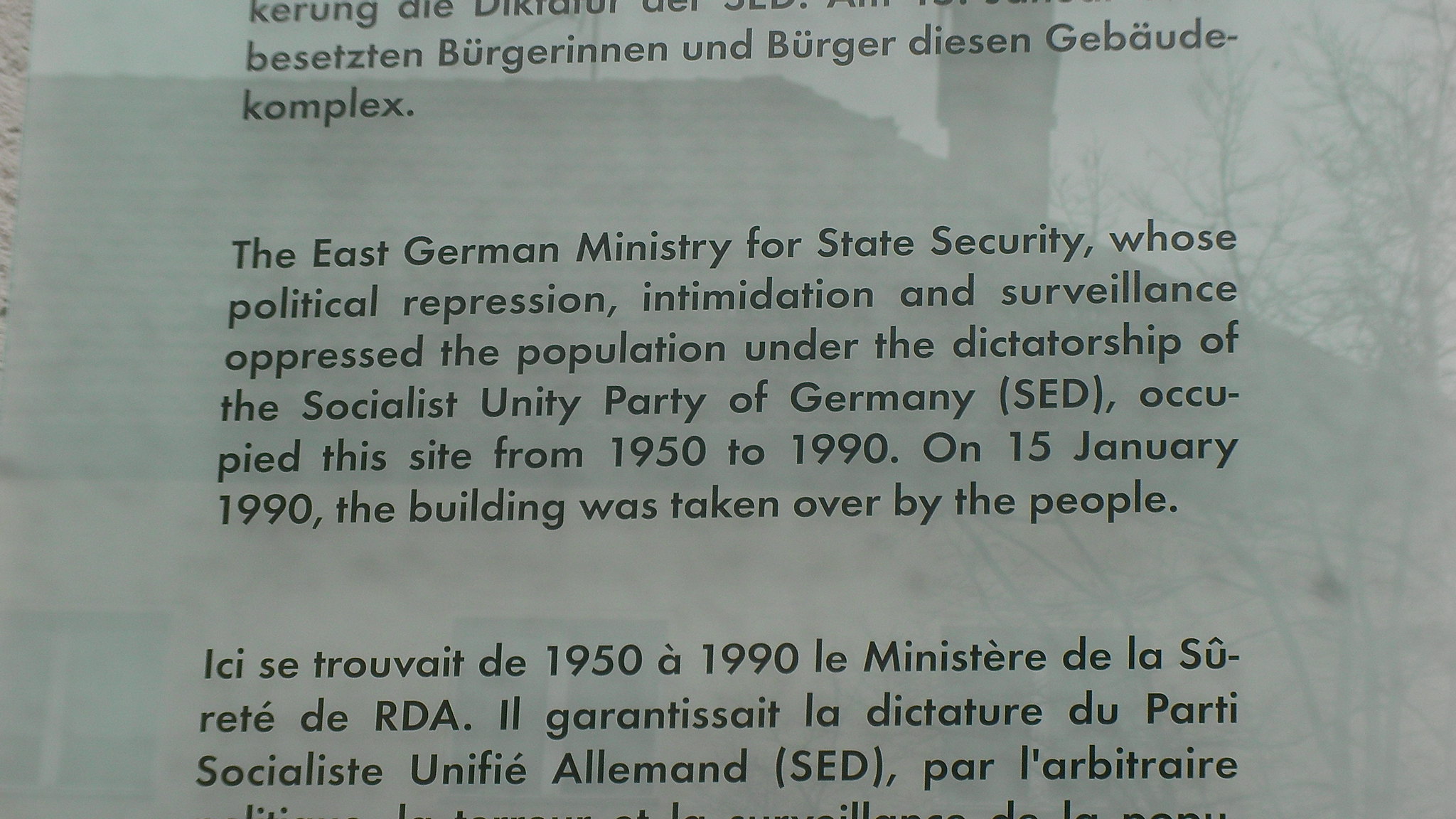The image depicts a close-up of a translucent, off-green plaque, possibly made of glass or plastic. The plaque is mounted on a surface, reflecting the background scenes of a building and bare tree branches. The text on the plaque is primarily in black, with the top portion written in German. The central part of the plaque features an English inscription, which reads: "The East German Ministry for State Security, whose political repression, intimidation, and surveillance oppressed the population under the dictatorship of the Socialist Unity Party of Germany (SED), occupied this site from 1950 to 1990. On 15 January 1990, the building was taken over by the people." Below this English text, there appears to be additional writing in French. The plaque, likely educational in nature, provides historical information about the building’s significance during East German rule.